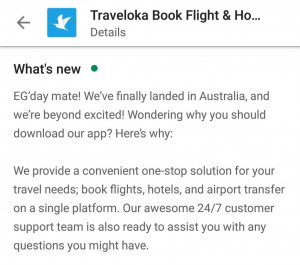A cell phone screenshot displaying the Traveloka app interface is captured. At the top of the screen, a white bird icon is prominently featured against a blue square background, representing the Traveloka logo. Immediately to the left of the logo, a back arrow icon is displayed, indicating the option to navigate to the previous screen. 

Directly below this, the header shows the text "traveloka traveloka book flight and HO..." followed by a "Details" button. A gray horizontal line spans the screen underneath this header. 

The next section is titled "What's New," highlighted by a blue dot adjacent to it. Below this heading, text reads: "EG-day mate," followed by an enthusiastic note, "EG-day mate! We finally landed in Australia and we're beyond excited! Wondering why you should download our app? Here's why:" 

Following this introduction, the content elaborates in a separate paragraph: "We provide a convenient one-stop solution for your travel needs: book flights, hotels, and airport transfers on a single platform." This is seamlessly followed by a note of assurance: "Our awesome 24/7 customer support team is also ready to assist you with any questions you might have."